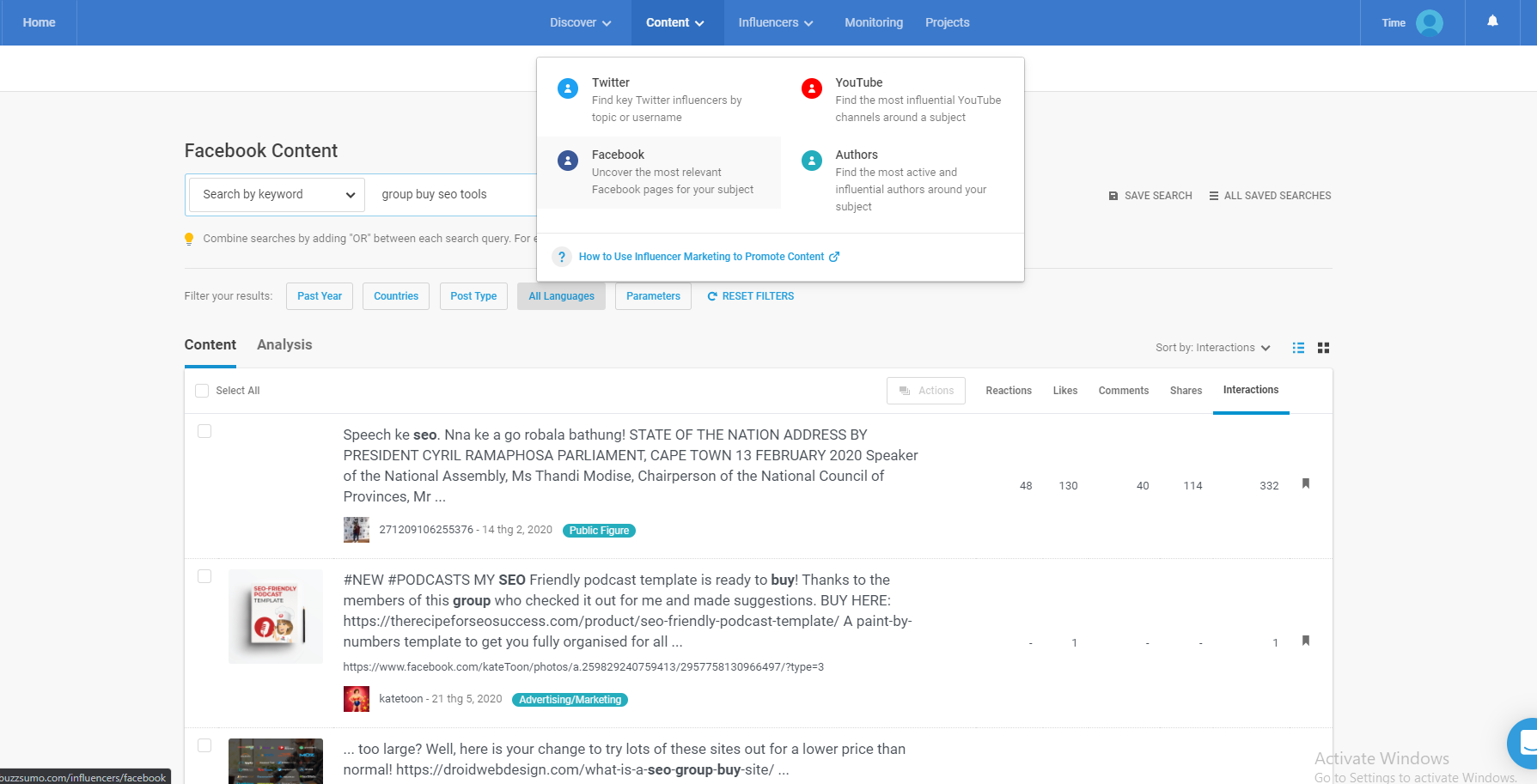This image captures a detailed screenshot of a computer screen focusing on a content management platform. 

### Description:

At the top, a blue bar menu spans the entire width of the screen. On the left-hand side, it features a "Home" button. Moving towards the center, the menu displays options like "Discover," "Content," "Influencers," "Monitoring," and "Projects." Towards the right, there's a "Time" label beside a blank person icon and an alarm bell icon.

The "Content" button is highlighted with a slightly darker blue rectangle, indicating that it has been selected. Below this, a popup menu displays options such as "Twitter," "Facebook," "YouTube," and "Authors." The user has selected "Facebook" from this menu.

In the main section beneath the popup, the screen displays a header titled "Facebook Content." This section allows search by keyword and grouping by SEO tools. There are various filter options for the past year, country, post type, all languages, and parameters, along with an option to reset these filters.

Below the filter options, there is a heading titled "Content and Analysis" indicating that the content has loaded. The first entry is labeled "Speech Key SEO," featuring a post about the "State of the Nation Address by President Cyril Ramaphosa, Parliament Cape Town," denoted as a public figure. 

The second entry showcases what appears to be an image of a book, with the title "New Podcast: My SEO Friendly Podcast Template is Ready to Buy." 

Finally, there is a partially visible third entry with an image cut off, accompanied by text that reads, "Too large? Well, here’s your change. You should try lots of these sites for a lower price than normal."

The overall image provides a thorough glimpse into how influencer marketing content is managed and analyzed through the platform.